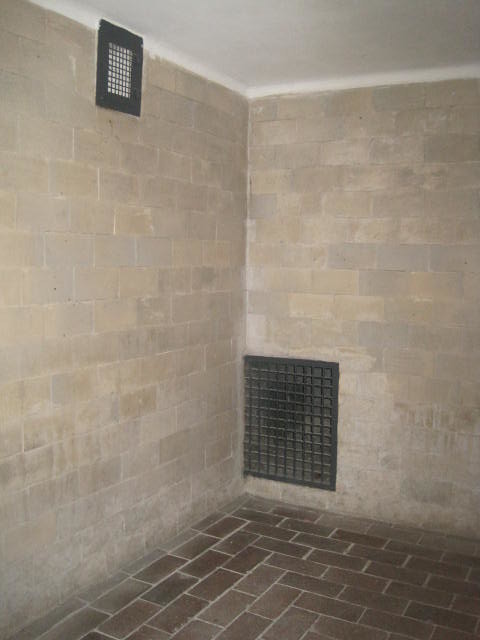The image presents a vertically aligned rectangle of an indoor setting, resembling a basement or crawl space. The room's corner showcases two intersecting brick walls and a brick-paved floor. The floor bricks are medium brown with light gray or white grout lines. The walls, in a contrasting shade, are paved with lighter brick material in tan beige and light gray tones. 

At the base of the right wall, centrally placed within the image, is a prominent dark brown or black vent grid, featuring a pattern of horizontal and vertical lines forming small squares. Additionally, an upper left-hand vent appears near the ceiling on the left wall, carrying a similar grid pattern but with a white backdrop. The ceiling, painted solid white, completes the composition, adding to the detailed and confined ambiance of the space.